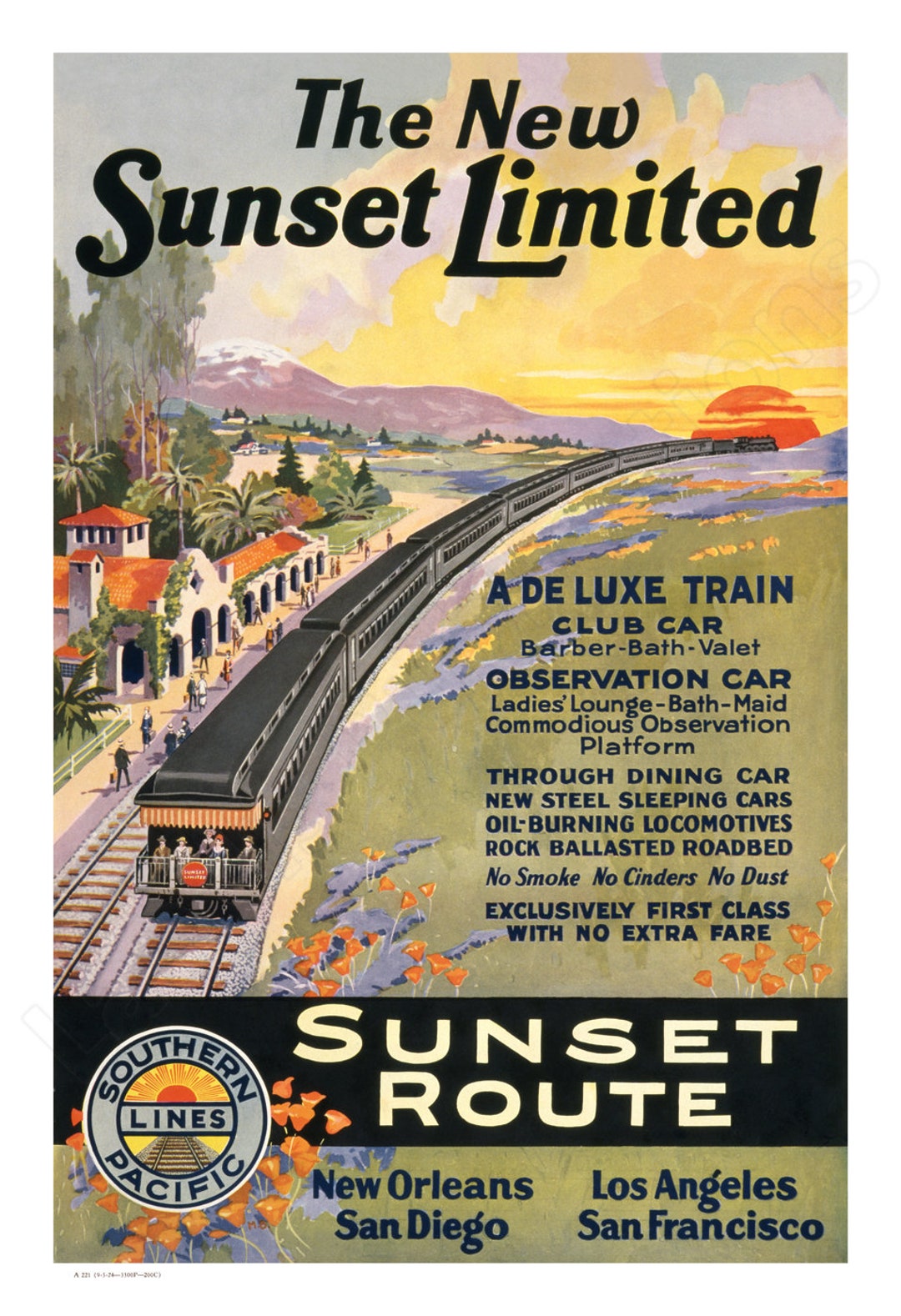This vividly illustrated poster promotes "The New Sunset Limited" train service. At the top, bold black text announces "The New Sunset Limited," while the right side of the middle lists the luxurious amenities: "a DELUXE train, club car, barber, bath, valet, observation car, ladies' lounge, bath, maid, commodious observation platform, through dining car, new steel sleeping cars, oil-burning locomotives, rock-ballasted roadbed. No smoke, no cinders, no dust, exclusively first class with no extra fare." The words "Sunset Route" are prominently displayed in white. At the bottom, the destinations "New Orleans, Los Angeles, San Diego, San Francisco" are listed, and to the left corner, it reads "Southern Pacific Lines."

Dominating the background is a beautiful painting of a train moving from the horizon towards the foreground, emerging from a large, red sun setting behind it. The sky is a gradient of yellow, pink, and blue, with lush grass and vibrant flowers on the right side of the train tracks. On the left side, a building with a red roof and white walls is visible, bustling with people walking towards the train. The picturesque scene is enriched with diverse colors, including green, orange, and purple, adding to the allure of this first-class travel experience.